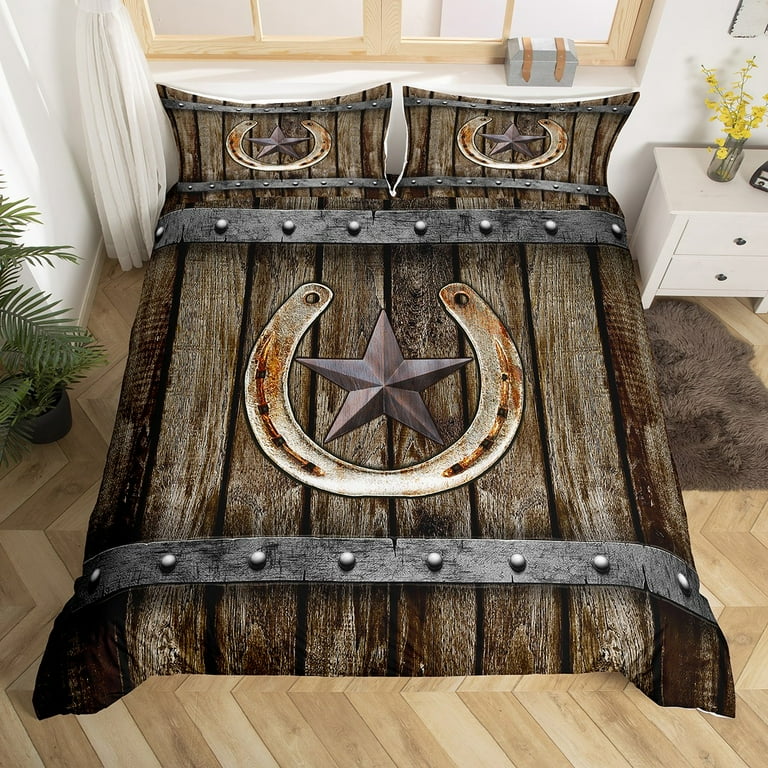This photograph, taken from a top-down perspective, captures the interior of a room with wooden flooring that features a light chevron pattern. In the center of the room stands a bed, covered with a brown bed sheet designed to look like an old rustic barn door. The bed sheet's design includes weathered wood, metal bands with rivets at the top and bottom, and a central horseshoe with a bronze star in the middle. Matching pillowcases carry the same aesthetic. To the right of the bed is a fuzzy brown rug and a white dresser with two drawers and a yellow potted plant on top. A vase with flowers is also situated on this side. Adjacent to the bed on the left is another potted green plant. The walls of the room are white, and above the bed is a window with curtains hanging down to the left. The overall decor evokes a barn-like aesthetic, with leather straps and a rustic ambiance.